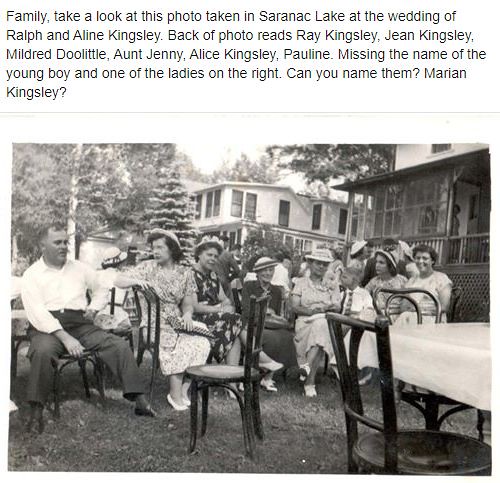This black and white photograph, taken at the wedding of Ralph and Aileen Kingsley in Saranac Lake, captures a nostalgic outdoor family gathering. The image shows a large group of people sitting at tables and chairs set up in a yard. Visible in the foreground is a man in dark pants and a white shirt, facing the camera, and a woman in a floral dress and hat turned towards him. Several other women, also dressed in calf-length, short-sleeved dresses and hats, are dotted throughout the scene, suggesting warm weather. Two white houses are prominently featured: one with a porch and latticework at its base in the midground, and a larger house fringed by various trees in the background. The annotated text at the top reads: “Family, take a look at this photo taken at Saranac Lake at the wedding of Ralph and Aileen Kingsley. Back of photo reads: Ray Kingsley, Jean Kingsley, Mildred Doolittle, Aunt Jenny, Alice Kingsley, Pauline. Missing the name of the young boy and one of the ladies on the right. Can you name them? Marion Kingsley?” This historical snapshot not only presents a moment of joy but also a mystery to be solved within the family lineage.